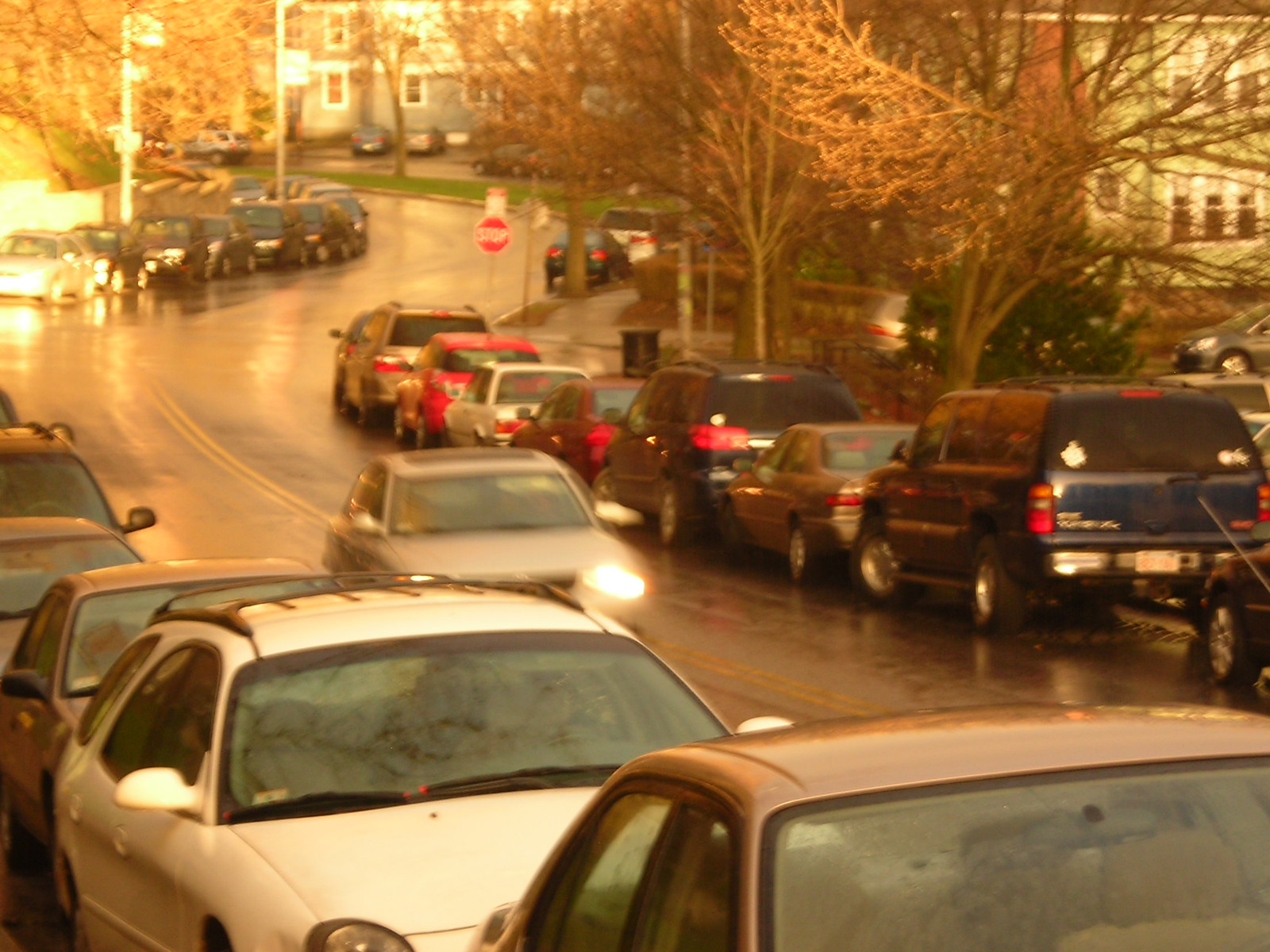This image depicts a bustling city street, seemingly captured during a busy rush hour shortly after a rain shower, as evidenced by the wet, shiny pavement and cars, coupled with the sunlight breaking through the clouds. The central focus is a four-way stop where an array of vehicles—approximately ten—are either lined up waiting or parked along the roadside. The road features two lanes in each direction, with cars traveling both towards and away from the camera. On the right-hand side of the image, a stop sign is prominently visible in front of the departing cars, which include various colors such as red, white, and blue. The incoming traffic includes a visible beige car and a white car, among others, following a curving path. The surrounding environment gives off an autumn vibe with barren trees and is contrasted by residential elements like houses with green lawns and driveways lining the street.